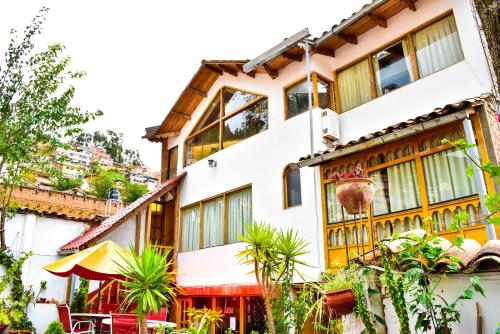This image depicts a stylized three-story home, possibly located in a tropical or desert-like area. The exterior features white plaster walls with yellow accents and orange-tiled roofs. The front of the house showcases several windows with distinctive blue and yellow curtains. The main structure is adorned with various architectural elements such as wide and thin supporting columns. On the first floor, there's a set of windows with yellow curtains pulled halfway down, and on the top floor, reflective windows display the open sky and surrounding trees.

The backyard reveals a serene outdoor setup with a white picnic table accompanied by red lawn chairs, all shaded by a yellow and white canopy. The background includes palm trees, a neighboring fence, and various desert or tropical plants, including some that resemble cacti. The sky appears overcast, adding a moodiness to the scene, while other homes and possibly mountains can be faintly seen in the distance.

A notable aspect is the detailed tile work on the various roofs, including a small peaked roof window that provides a panoramic view. The house also has a distinctive tri-level deck with arched wooden railings. The lower level, painted red, features porch doors opening to the backyard, while the second and third levels exhibit additional windows and a deck with arched fencing. Overall, the house's intricate details and vibrant colors contribute to its unique and artistic aesthetic.